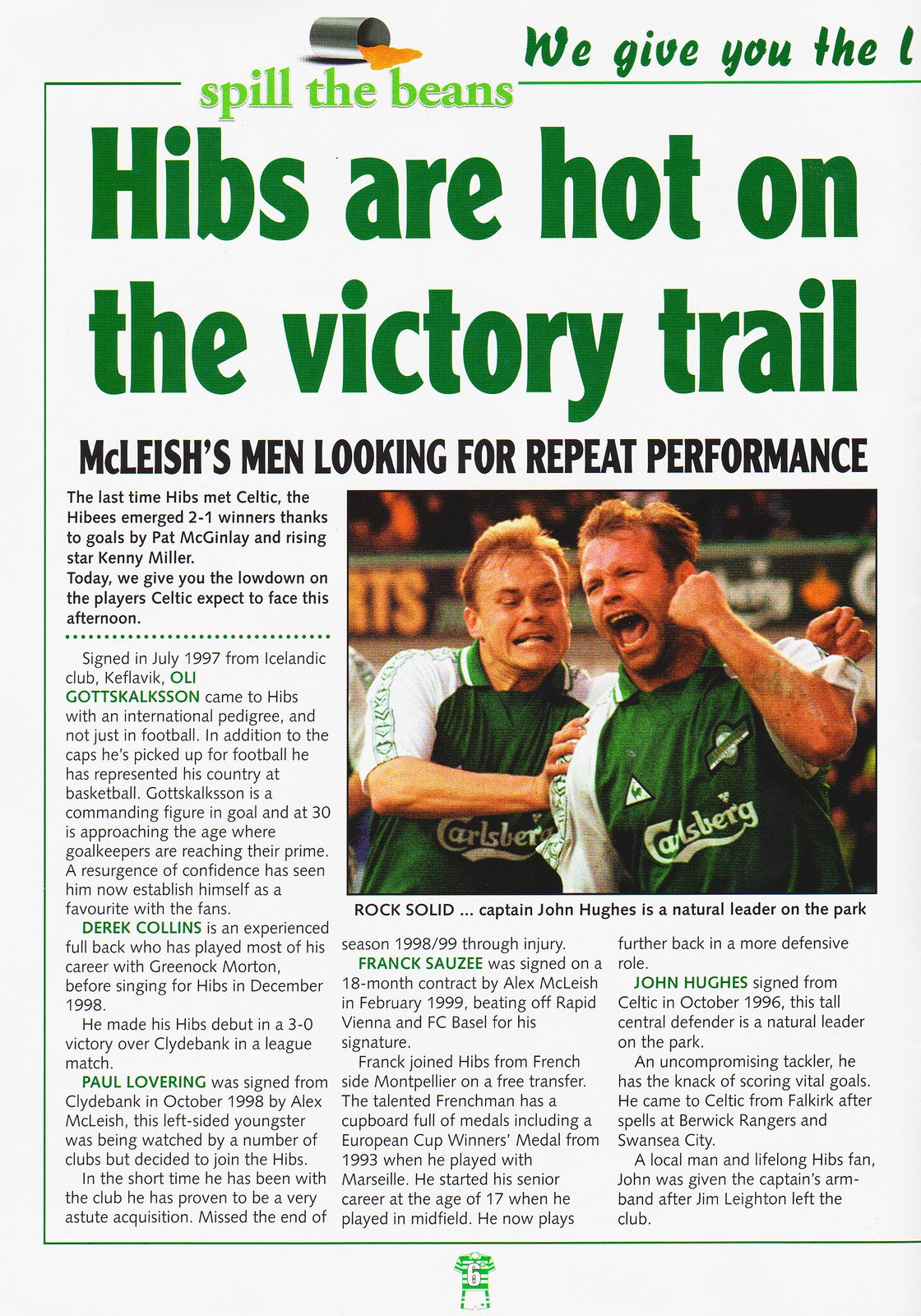This image features a partial magazine article with a white background and distinctive green text. Dominating the top is the headline, "We Give You the...", though the rest is obscured. Beneath this, in lime green, it reads "Spill the Beans" next to an illustration of a spilled can of beans. Prominently, the headline "Hibbs are Hot on the Victory Trail" stands out, followed by the subheading in black, "McLeish's Men Looking for Repeat Performance." The article starts with a description of a past match where the Hibbs triumphed 2-1 against Celtic, thanks to goals by Pat McKinlay and rising star Kenny Miller. It promises today's lowdown on the players Celtic will face, mentioning Olly Gottskalkson, signed in July 1997 from the Icelandic club Keflavik, among others. Each player’s name, including Derek Collins, Paul Lovering, Frank Sauzée, and John Hughes, appears in green, while the rest of the text is black. A photo captures two soccer players in green and white Carlsberg jerseys, either cheering or intensely engaged in play, with the caption noting "rock-solid Captain John Hughes is a natural leader on the park." Page six is indicated by a green and white uniform's image.